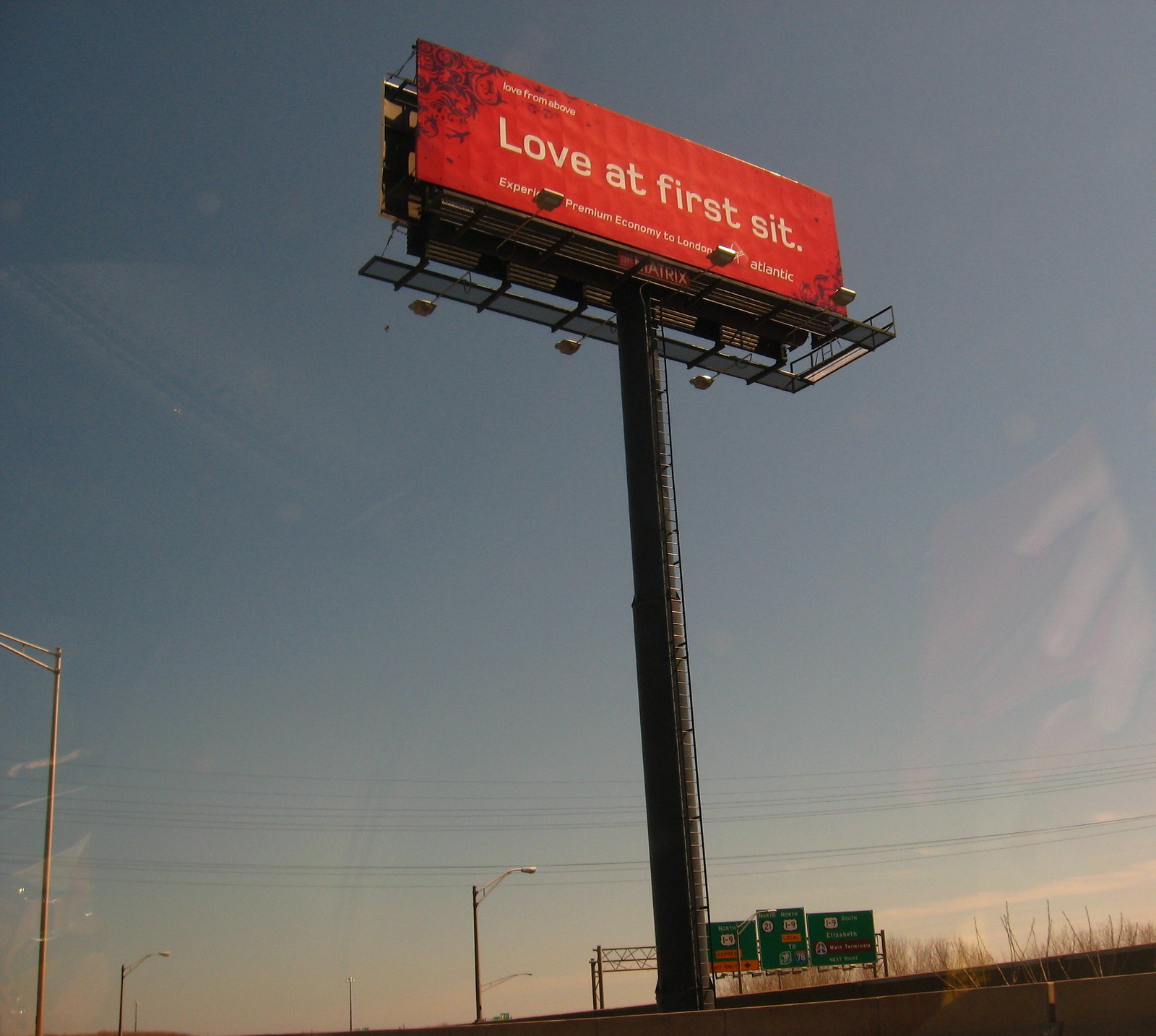The image showcases a very tall billboard photographed from ground level, emphasizing its towering presence. The billboard has a striking red background with bold white text that reads "Love at First Sit." This advertisement promotes Atlantic's premium economy service to London, and their symbol is visible on the right side of the billboard. The billboard is mounted on a thick metal pole equipped with a ladder extending down the front, while metal platforms with lights protrude from either side, illuminating the sign.

In the background, another billboard is faintly visible to the left. The sky is a clear blue with sparse clouds, indicating late afternoon or early evening, as dusk begins to settle. At the bottom of the pole, multiple green road signs provide directions, hinting that this towering advertisement is located near a bustling highway. Although the text on these signs is not entirely clear, they suggest routes including I-9, North 21, South 21, and 76. Surrounding the scene, there are some tree branches and traffic lights, further illustrating the highway setting.